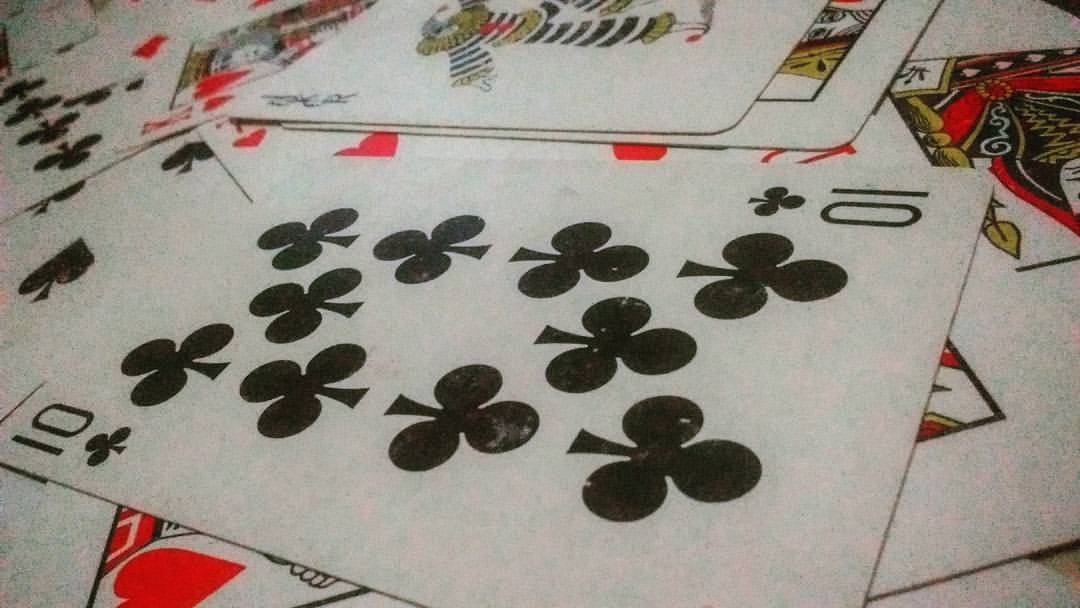A scattered deck of playing cards is spread across a table, completely covering its surface. The most prominent card in the foreground is the ten of spades. Behind it, partially visible, is a black Joker card. To the right, there appears to be a black face card, possibly a king or queen. In the background to the left, the red king card can be seen peeking out from beneath the spread. The table underneath is entirely concealed by the assortment of cards.